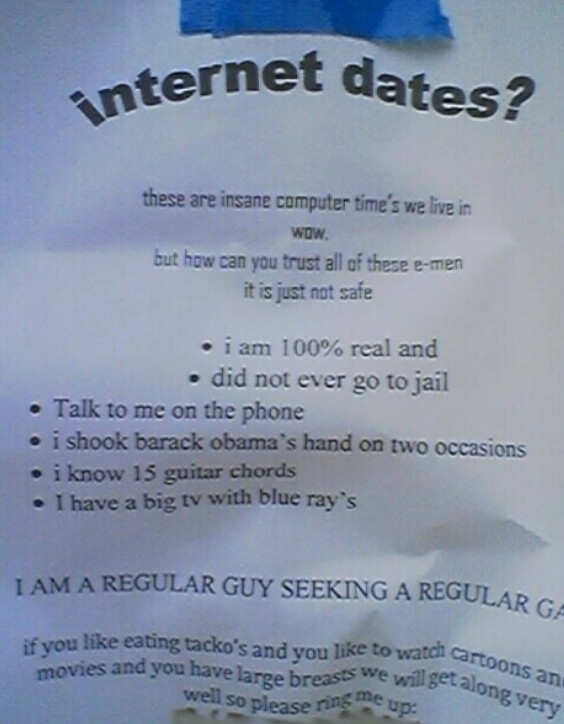This image is an advertisement for an online dating site, depicted on a crumpled piece of paper with a light blue background and some white at the top. Blue cloth is visible beneath it. The text, all in black, starts with a bolded and curving "Internet dates?" followed by the phrases "These are insane computer times we live in. Wow! But how can you trust all of these e-men? It is just not safe." Below this, a series of bullet points lists various personal attributes: "I am 100% real," "Did not ever go to jail," "Talk to me on the phone," "I shook Barack Obama's hand on two occasions," "I know 15 guitar chords," and "I have a big TV with Blu-rays." At the bottom, it states in all caps, "I am a regular guy seeking a regular gal. If you like eating tacos (spelled T-A-C-K-O-S), watching cartoons and movies, and you have large breasts, we will get along very well. Please ring me up," followed by a redacted phone number. The overall tone questions the safety of online dating while presenting a humorous and somewhat unconventional personal ad.